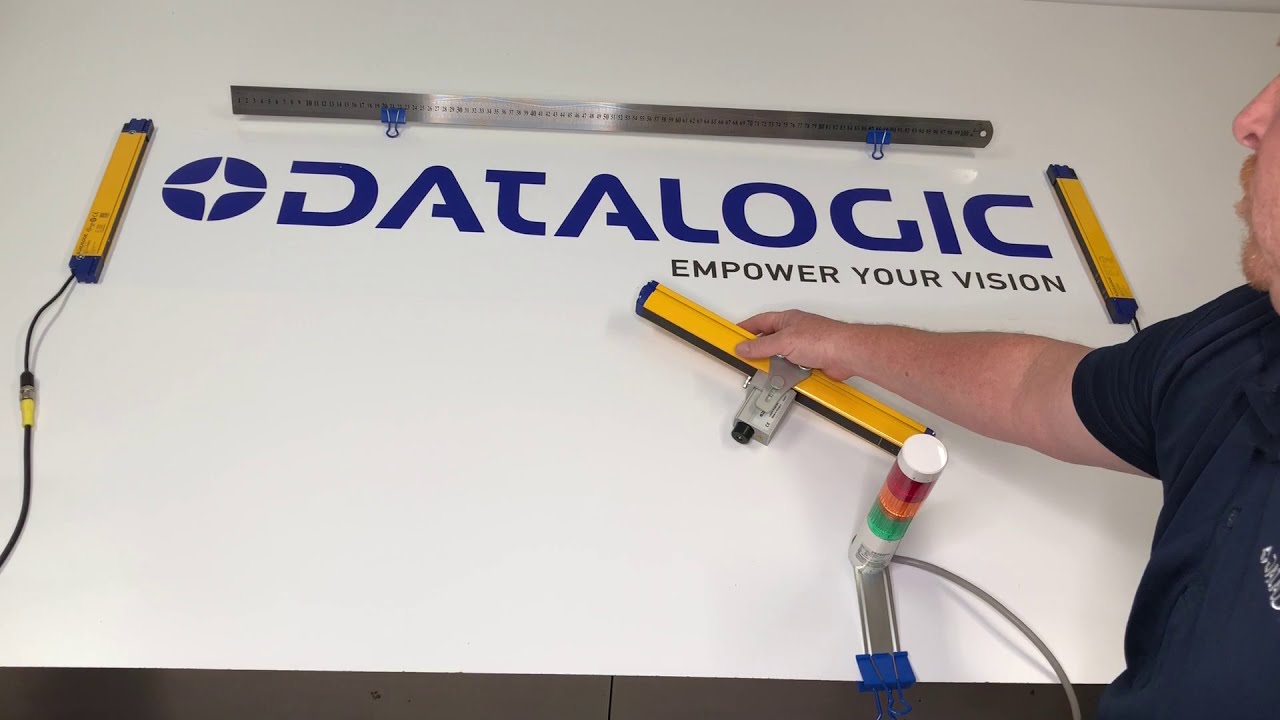In this image, a man stands in the bottom right corner, wearing a navy blue short-sleeved t-shirt. He appears to be Caucasian with pale skin and reddish-orange hair, although his face is not fully visible. His hands are holding a yellow measuring tool with black accents and a silver device attached, pressing it against a white surface. The man seems to be working with what might be a level or stud finder. 

The central focus of the image is a blue-font “Datalogic” logo with an adjacent circle featuring a yellow cross resembling a Phillips head screw. Below the logo, the phrase "EMPOWER YOUR VISION" is written in black capital letters. There are additional yellow measuring tools, similar to the one the man is holding, positioned on either side of the logo with cords connected to them. Above the logo is a metal object that looks like a metal ruler with clips attached. The colors in the image include white, yellow, blue, silver, and orange, suggesting the setting may be a workplace environment or part of an advertisement.